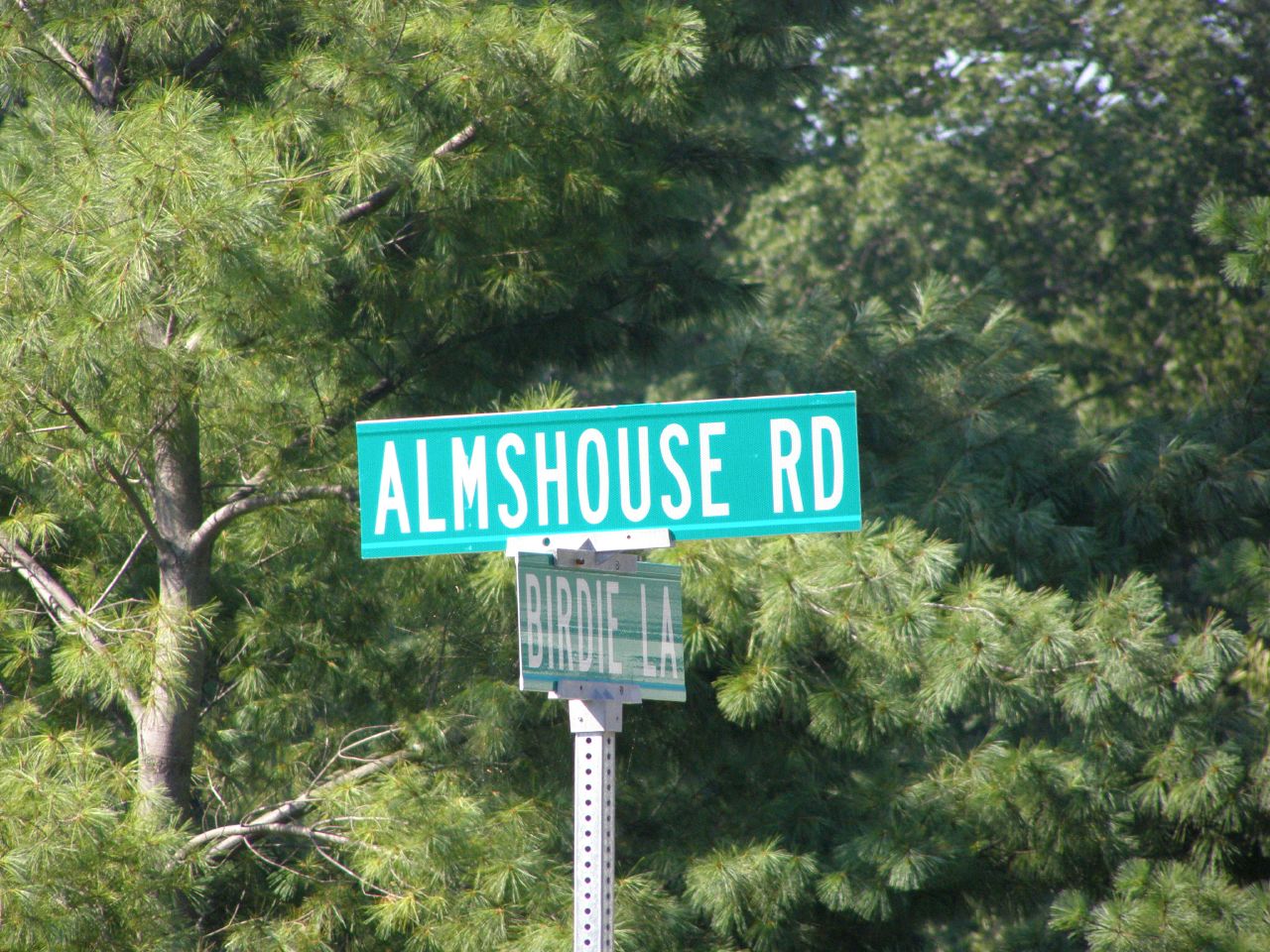This color photograph captures a detailed view of a street sign mounted on a square-shaped, silver metallic pole perforated with small holes. The image features two green rectangular signs with white lettering: the top sign reads "Almshouse Road," while the sign below it indicates "Birdie, LA." The scene is set against a verdant backdrop of green conifer trees, possibly pines, through which patches of blue sky are faintly visible. Bright sunlight illuminates the scene, casting varied shadow patterns within the lush green foliage, highlighting both darker and lighter shades of green. The photograph is taken from a side perspective, showcasing approximately a foot of the metallic pole that supports the signs.